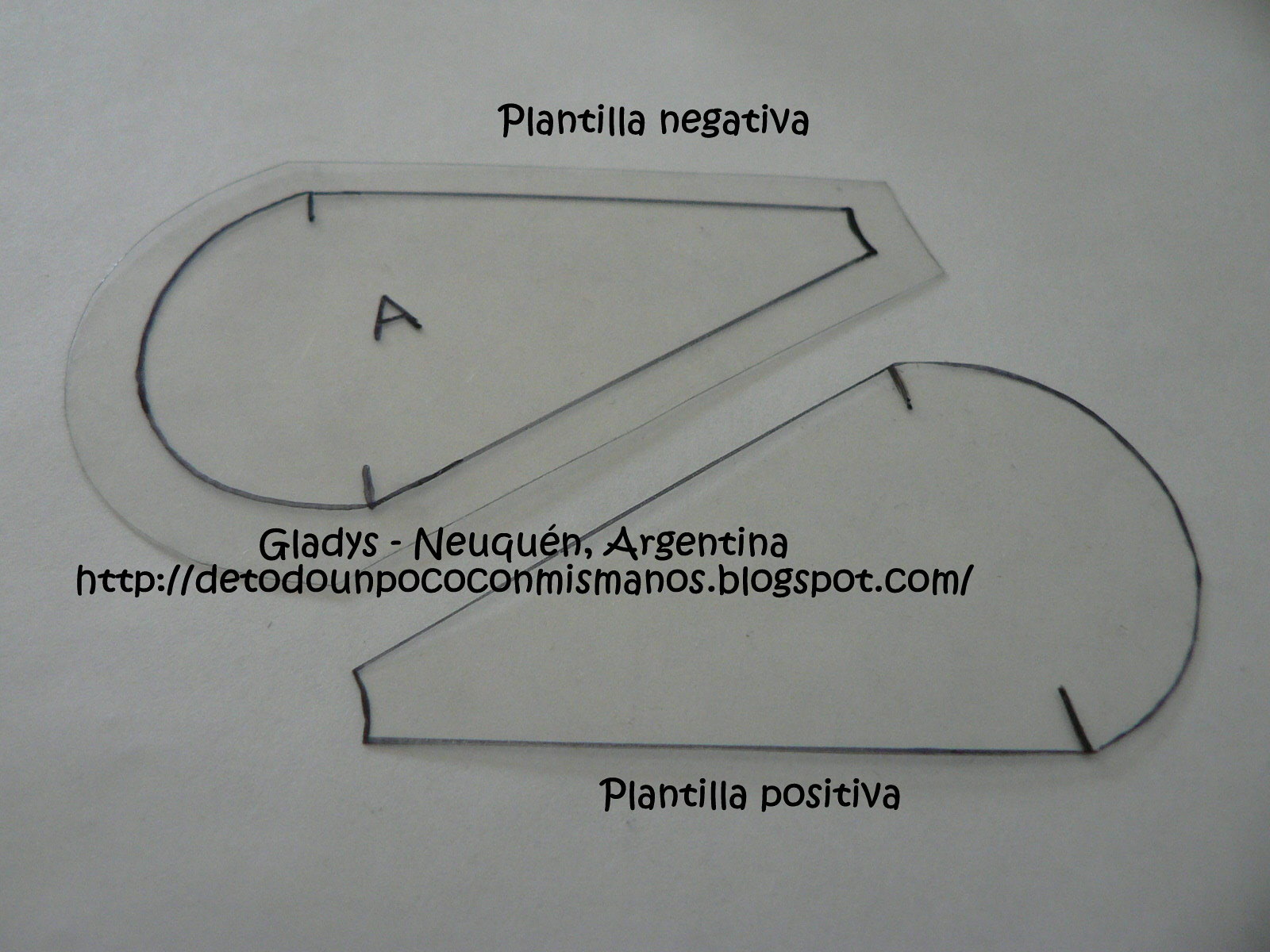The image depicts a computer-generated drawing on a white background, resembling a piece of paper. At the very top center, the text reads "Plantilla Negativa." Below, there are two outlined shapes that resemble ice cream cones or parachutes, drawn with black lines. The top shape contains the letter "A" in its middle. In the center of the image, the black text reads "GLaDOS, Nequen, Argentina, Plantilapositiva.com." Towards the right-hand side, beneath the other shape, which is similarly designed but without additional markings, the text "Plantilapositiva" can be seen. Additionally, a web address "HTTP://DTO.donpocomisamos.blogspot.com" is also mentioned.